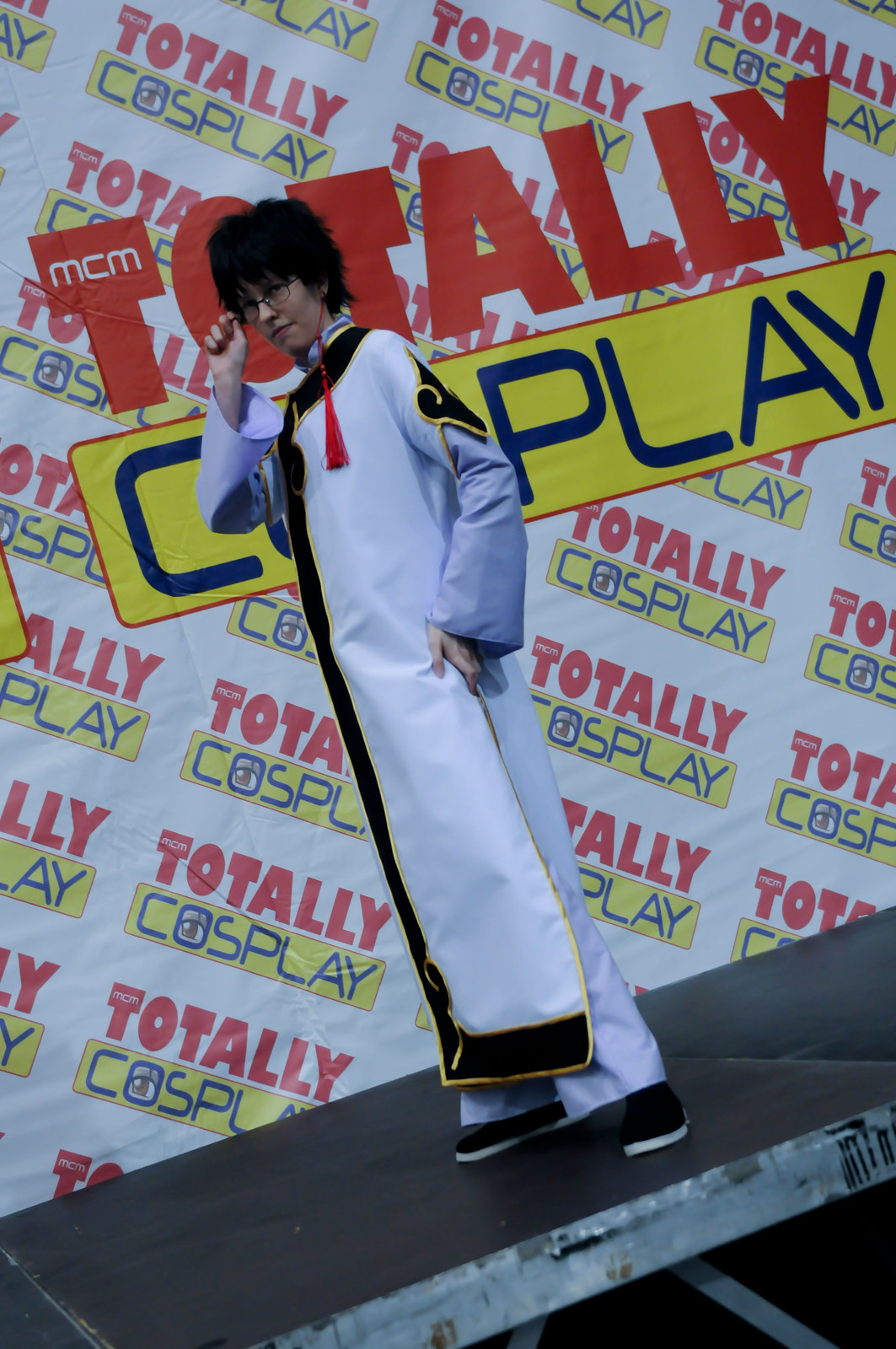The photograph features a person posing on a stage platform in front of a repeating backdrop that reads "Totally Cosplay," with "Totally" in bold red letters and "Cosplay" in bold blue letters, all set on a yellow rectangular background. The individual stands on a black surface flooring, wearing a long white coat with black piping, white pants, and black shoes. The coat, which possibly resembles priest attire, also features black and gold designs, including a black symbol that looks like a fleur-de-lis on one sleeve. The person has jet-black shaggy hair, is wearing black glasses, and is depicted with one hand up, touching their glasses. A noticeable detail is their red tassel earring hanging in front of the coat. The overall color palette of the image includes red, blue, yellow, white, and black.